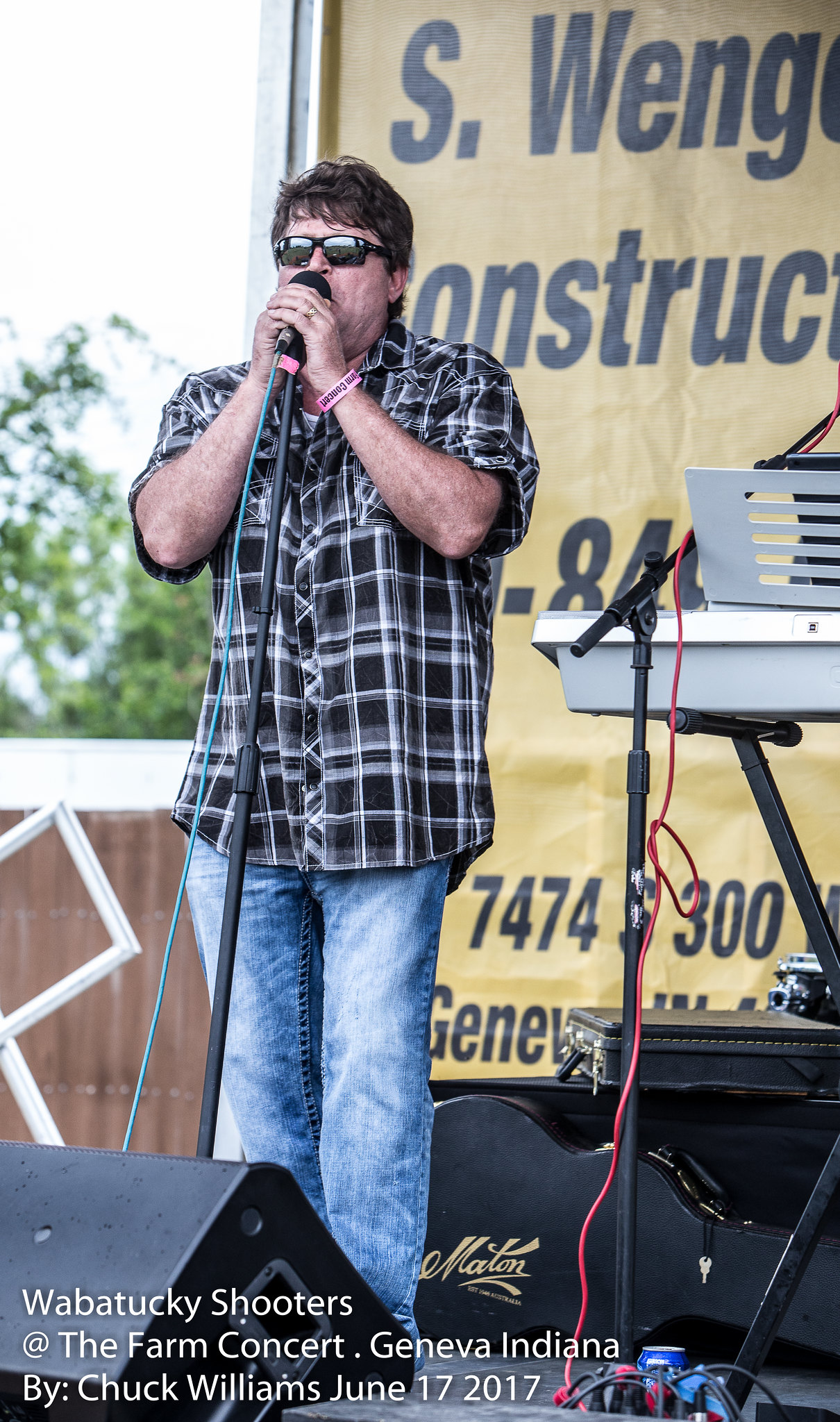This is a detailed photograph of a male performer on stage during the Wabatuckee Shooters concert at the Falmerham Concert, Geneva, Indiana, on June 17, 2017, as noted in the watermark by Chuck Williams at the bottom left corner. The singer, a white man with shaggy, medium-length brown hair, is wearing black shades and a short-sleeved black and white plaid button-up shirt paired with light blue jeans. He grips the microphone stand with both hands as he passionately sings. Behind him, a partially visible sign, possibly an advertisement with cut-off text, serves as a backdrop. To the right, just out of full frame, a keyboard stands, while a guitar case with the logo for Matten lies behind the singer's legs, further indicating the musical setting.